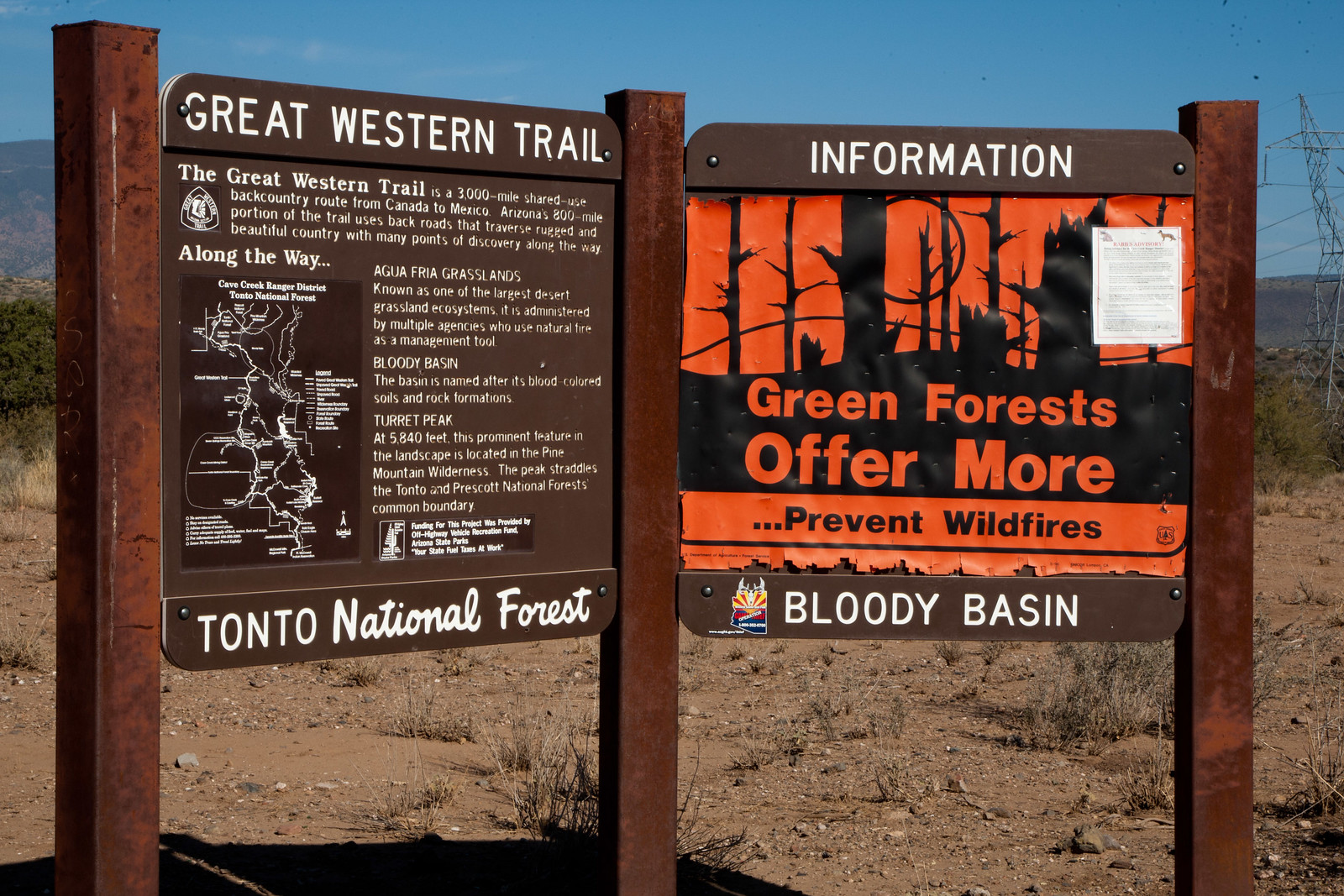This image captures two vertically rectangular signs situated next to each other, set against a backdrop of brown dirt, low grass, and some hills, all under a clear blue sky. Each sign is mounted on a pair of dark brown wooden posts, and they share a center post. The left sign displays the title "Great Western Trail" and "Tonto National Forest," providing a detailed map and trail information. The map highlights the 3,000-mile backcountry route and points out notable sites like the Bloody Basin. The right sign features a combination of text and imagery; at the top, it states "information." Lower down, it reads "Bloody Basin" in white text with an orange and black visual representation where the orange represents fire, and the black depicts barren, leafless trees, emphasizing fire prevention with the message, "Green forests offer more, prevent wildfires." A small, unreadable white piece of paper is also attached to the right sign. In the background, power lines and a transformer tower are visible, reinforcing the rustic yet managed setting.